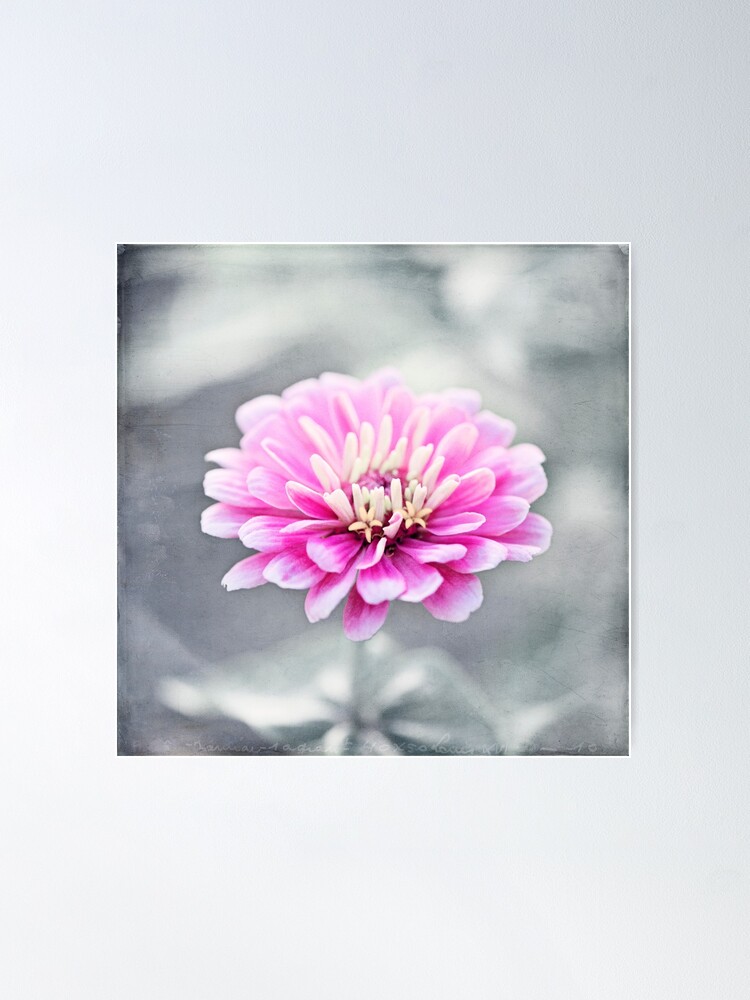The image is a detailed and elegant depiction of a pink flower that appears to be rendered in a watercolor-like style. The flower is characterized by its numerous layers of thick, intricately arranged petals, which radiate a soft pink hue with subtle purple undertones. At the heart of the bloom are striking white, stem-like growths that add to its allure. The background is a gray and white, blurry canvas with brushstroke textures, enhancing the vividness and beauty of the flower. The entire composition is framed by a faint gray border, lending an almost photographic quality to the piece, despite its painterly elements. The harmonious blend of colors and textures draws attention to the flower's delicate details, making it the focal point of the image. There is also a faint, unreadable text at the very bottom of the piece, adding a subtle, mysterious touch.